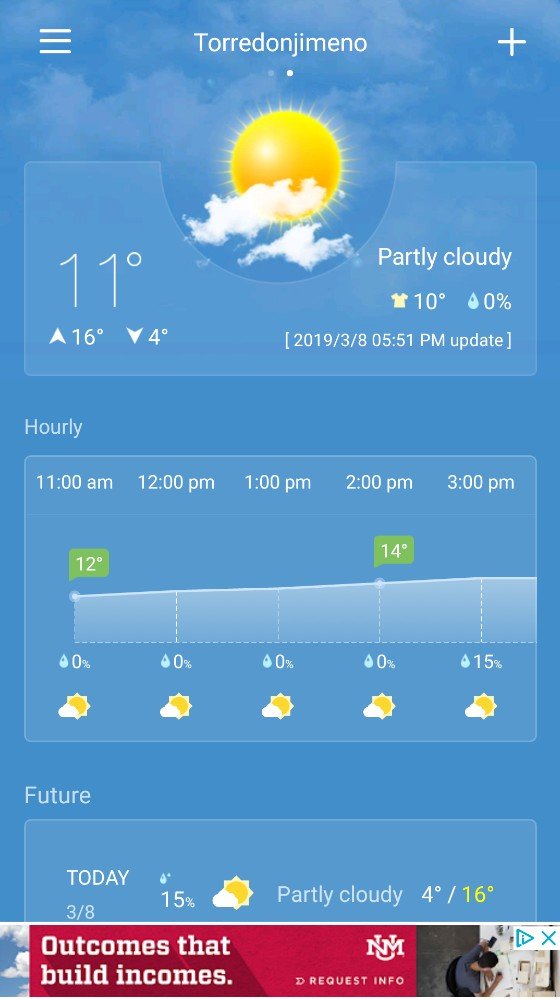Here is the cleaned-up and detailed caption for the image:

---

The image is a screenshot of a weather app taken on a cell phone. At the top of the screen, there is a hamburger menu on the left and a plus sign on the right, likely for adding additional locations. Currently, the page displays weather information for Torredonjimeno. Below the menu, there are two dots, with one highlighted, indicating that there are two saved locations that can be accessed by scrolling.

The main section of the screen shows that the weather in Torredonjimeno is partly cloudy, depicted by an icon of the sun with a few clouds. The current temperature is 11 degrees Celsius, with a forecasted high of 16 degrees and a low of 4 degrees. A shirt icon next to the number 10 suggests a "feels like" temperature of 10 degrees Celsius. The precipitation probability is shown with a raindrop icon and 0%, indicating no chance of rain. The last update was on March 8, 2019, at 5:51 p.m.

Below this information is an hourly forecast displaying the temperature and chance of rain throughout the day. The temperatures range from 12 to approximately 15 degrees Celsius, with specific labels showing 12 degrees at 11 a.m. and 14 degrees at 2 p.m.

The final section, labeled "Future," provides an additional forecast for the day, showing a 15% chance of rain, partly cloudy skies, and temperatures ranging from 4 to 16 degrees Celsius.

At the bottom of the screen, there is a banner advertisement featuring the slogan "Outcomes that build incomes" and a logo featuring the letters "NM" on top of a "U." This might suggest an affiliation with New Mexico University, although it is not explicitly stated.

---